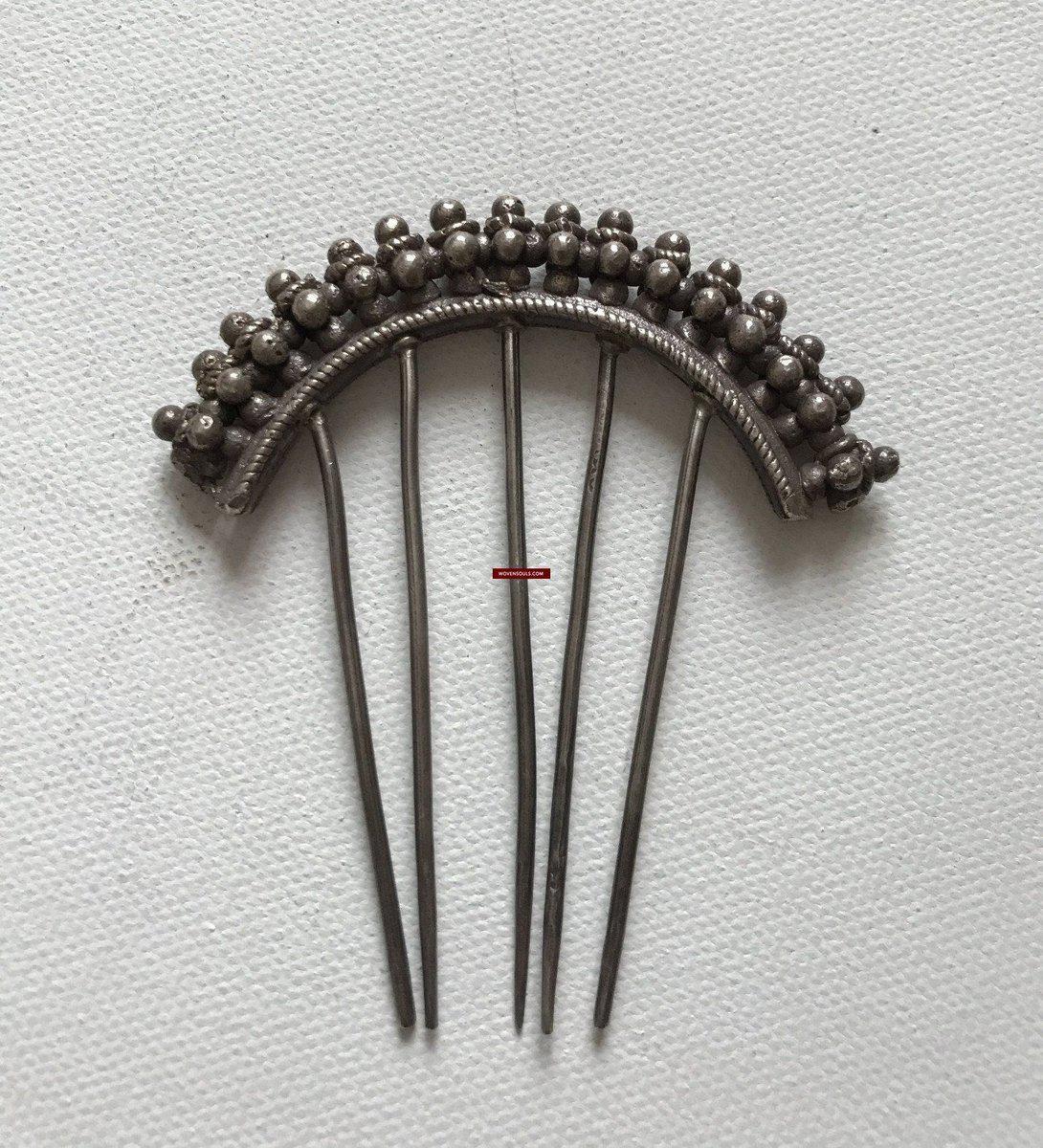This is a detailed photograph of a vintage hairpin made of tarnished silver or dull bronze metal with a pewter-like appearance. The hairpin features a distinctive arch-shaped top adorned with small, round orbs that resemble metal pearls or beads, forming a decorative pattern with three columns of beads laying next to each other across the arch. Beneath the arch hang five long, slender prongs that suggest its use as a hair accessory. Positioned at the center of the arch is a tiny red rectangle with small, illegible white text. The hairpin rests on a textured white surface that resembles a paper towel or napkin, which appears slightly dirty with visible lines and black specks.